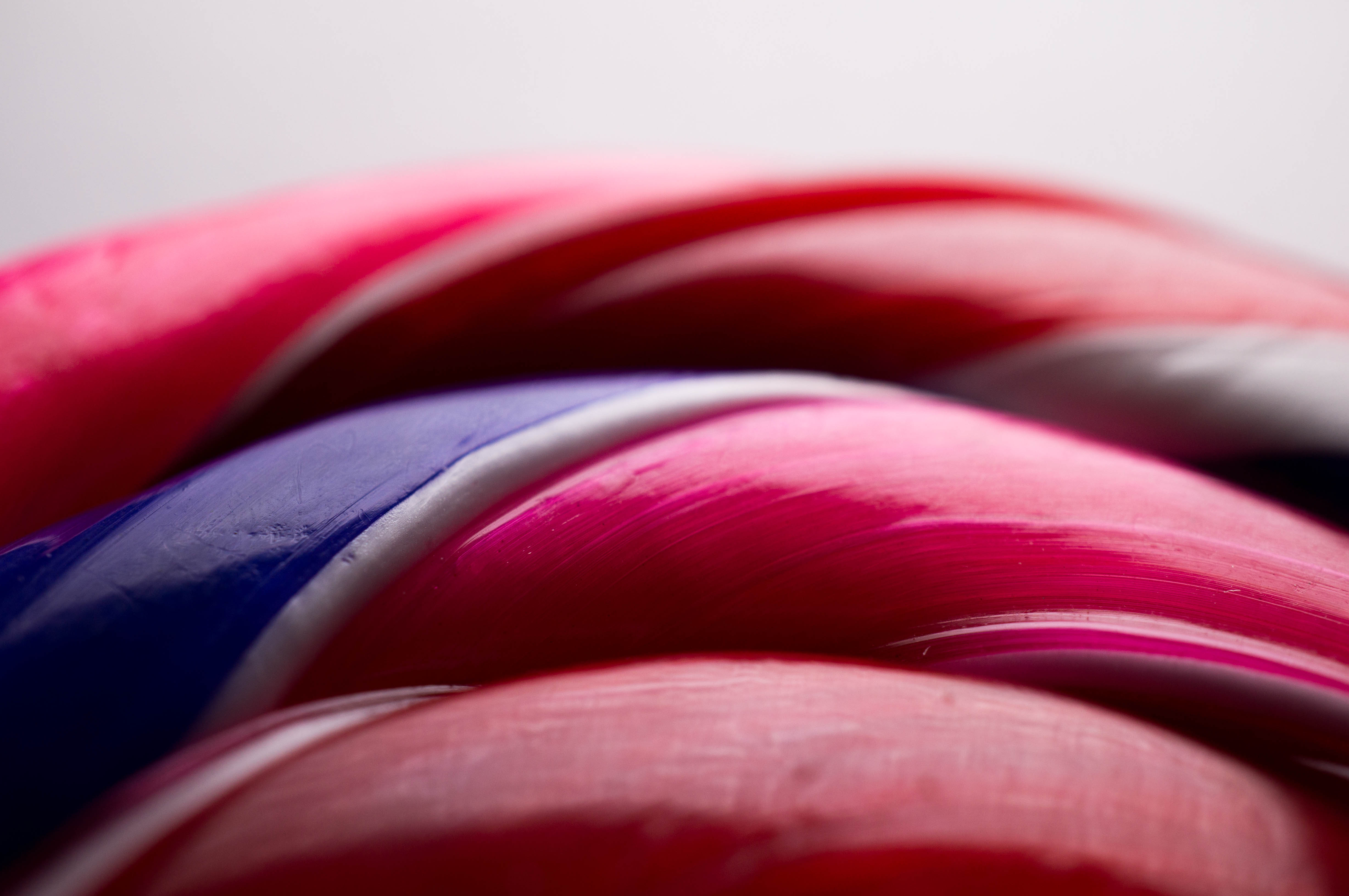This photo captures three twisted, curved objects, closely situated and nearly touching, taking up about three-quarters of the frame both horizontally and vertically. Primarily red in color, these objects have a glossy sheen that suggests a candy-like texture, reminiscent of saltwater taffy. One of the objects, specifically on its left edge, features blue and white coloring, adding to the impression of colorful confectionery. Their shiny and slightly bent appearance strengthens the resemblance to traditional taffy. The background showcases a plain white surface, which could either be a wall or a table, providing a clean and simple contrast to the vivid hues and intricate twists of the objects in the foreground.